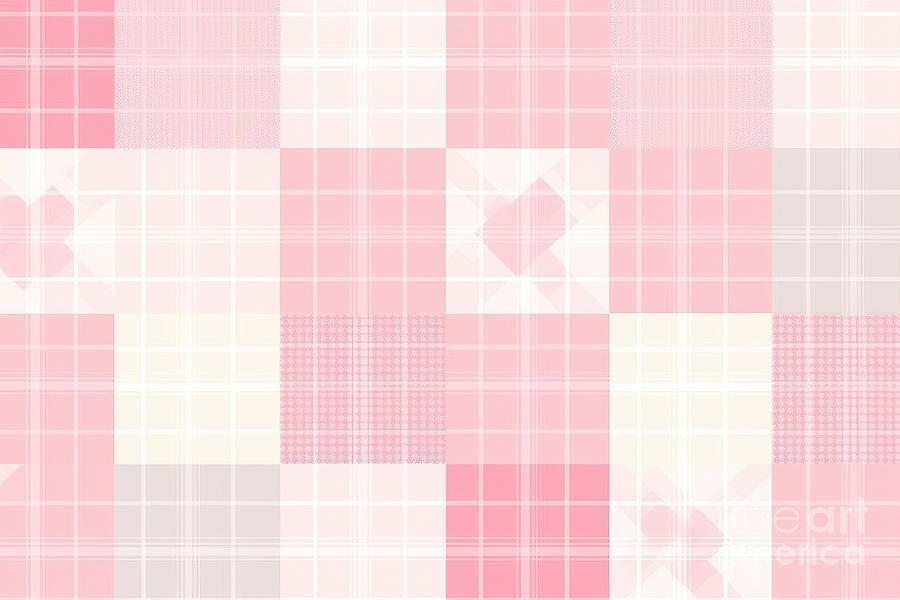This image depicts a digitally created artwork featuring an intricate and complex pattern of squares arranged methodically on a canvas. The squares vary in shades predominantly of pink and red, interspersed with hues of gray, white, and even some that could be perceived as beige or yellow. The pattern resembles a net, with white lines crisscrossing the squares, reminiscent of a soccer net. Each square is meticulously placed, with varying tones creating a visually appealing gradient effect; for example, the top left has a dark pink square followed by progressively lighter shades of pink.

There's faint text overlaying the image at the bottom, possibly a watermark, that is difficult to read. In the bottom right corner, a transparent image or watermark subtly blends into the artwork, indicating some form of branding or signature.

The detailed arrangement of approximately 300 squares suggests the image could serve as a decorative element, perhaps for Valentine's Day cards, given its romantic pink and red palette. The deliberate and elegant composition of shapes and colors showcases a high level of artistry and digital craftsmanship.